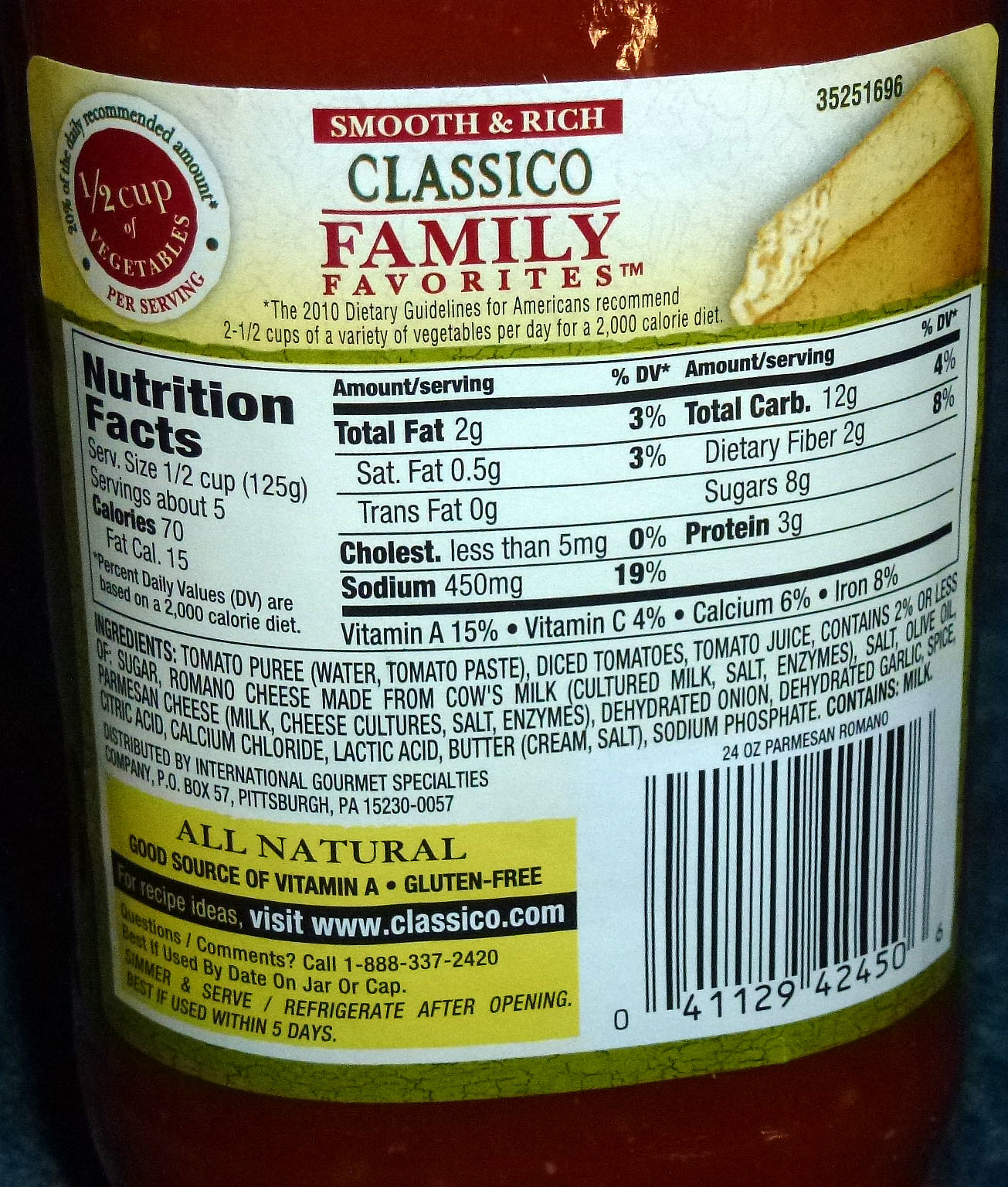This is a close-up photograph of the back of a 24-ounce jar of Classico Parmesan Romano pasta sauce, clearly focusing on its detailed nutritional label. The glass bottle showcases a hint of the rich red sauce inside, but the main focus is the label. At the top, the label prominently features the brand's tagline, "Smooth and Rich Classico Family Favorites," set within a green-bordered white section, adorned by a half-cut wheel of Parmesan cheese.

To the side, in a round red circle, it highlights that each serving contains "half a cup of vegetables." The nutritional facts panel is extensive, detailing a serving size of half a cup (125 grams), with about five servings per container. It lists the exact nutritional values: 70 calories per serving, 2 grams of total fat, 0.5 grams of saturated fat, 0 grams trans fat, under 5 milligrams of cholesterol, 450 milligrams of sodium, 12 grams of total carbohydrates, 2 grams of dietary fiber, 8 grams of sugars, and 3 grams of protein. Additional nutrient information includes 15% Vitamin A, 4% Vitamin C, 6% Calcium, and 8% Iron.

Below the nutritional facts, the ingredients are meticulously listed: tomato puree (water, tomato paste), diced tomatoes, less than 2% of sugar, Romano cheese (cow's milk, cultured milk, salt, enzymes), salt, olive oil, Parmesan cheese (milk, cheese cultures, salt, enzymes), dehydrated onion and garlic, spices, citric acid, calcium chloride, lactic acid, butter (cream, salt), and sodium phosphate. The product contains milk and is distributed by International Brody Specialties Company, based in Pittsburgh, PA.

On the lower section of the label, to the right, there is a barcode, while to the left, in a yellow rectangle, it states "All-natural, Good source of Vitamin A, Gluten-free." For recipe ideas, the label suggests visiting www.classico.com, and provides a customer service phone number: 1-888-337-2420. The label also includes usage instructions, advising to simmer and serve, refrigerate after opening, and consume within five days for best quality.